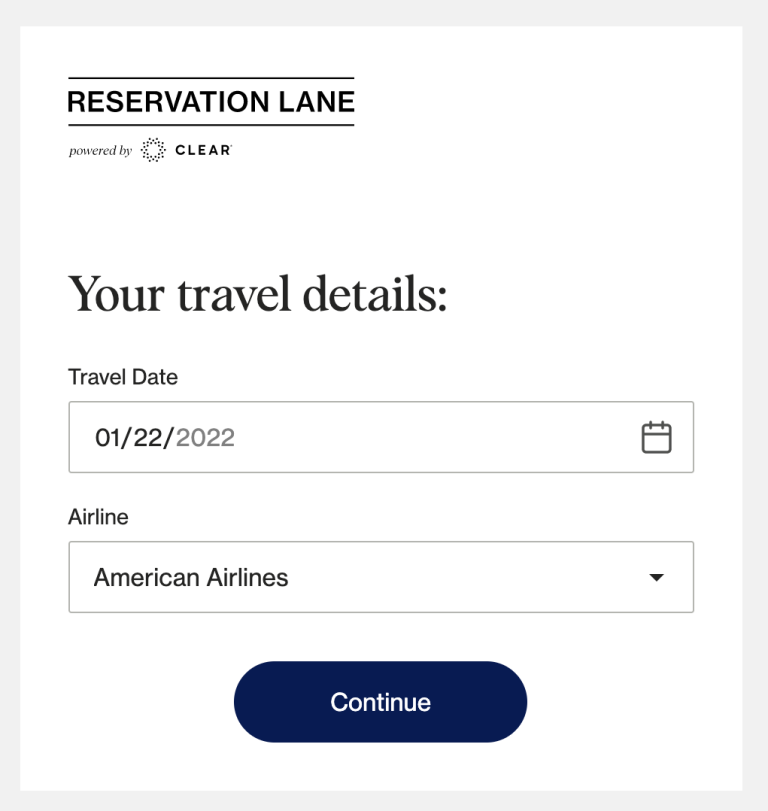The image is a square web graphic featuring a clean, minimalist design against a white background. It is bordered by a very light gray, thin border. In the upper left-hand corner, there is a prominent header "RESERVATION LANE" in capital letters, flanked above and below by thin black lines. Just below this, in a smaller italic font, the phrase "Powered By" is displayed next to a distinctive star logo formed with dots. To the right of the star logo, "CLEAR" is written in bold black, capitalized text. 

Centrally placed, a larger and differently styled text reads "Your Travel Details." Below this heading, two labeled input boxes are neatly arranged: the "Travel Date" box, identified by a small calendar icon on its far right, shows the entered date "01/22/2022," and the "Airline" box, a drop-down menu, indicates "American Airlines" as the selected option. Both input boxes are enclosed with a thin gray line, giving a structured look.

At the bottom center of the graphic is a wide, dark navy blue button, prominently displaying "CONTINUE" in crisp white text at its center, inviting user interaction.